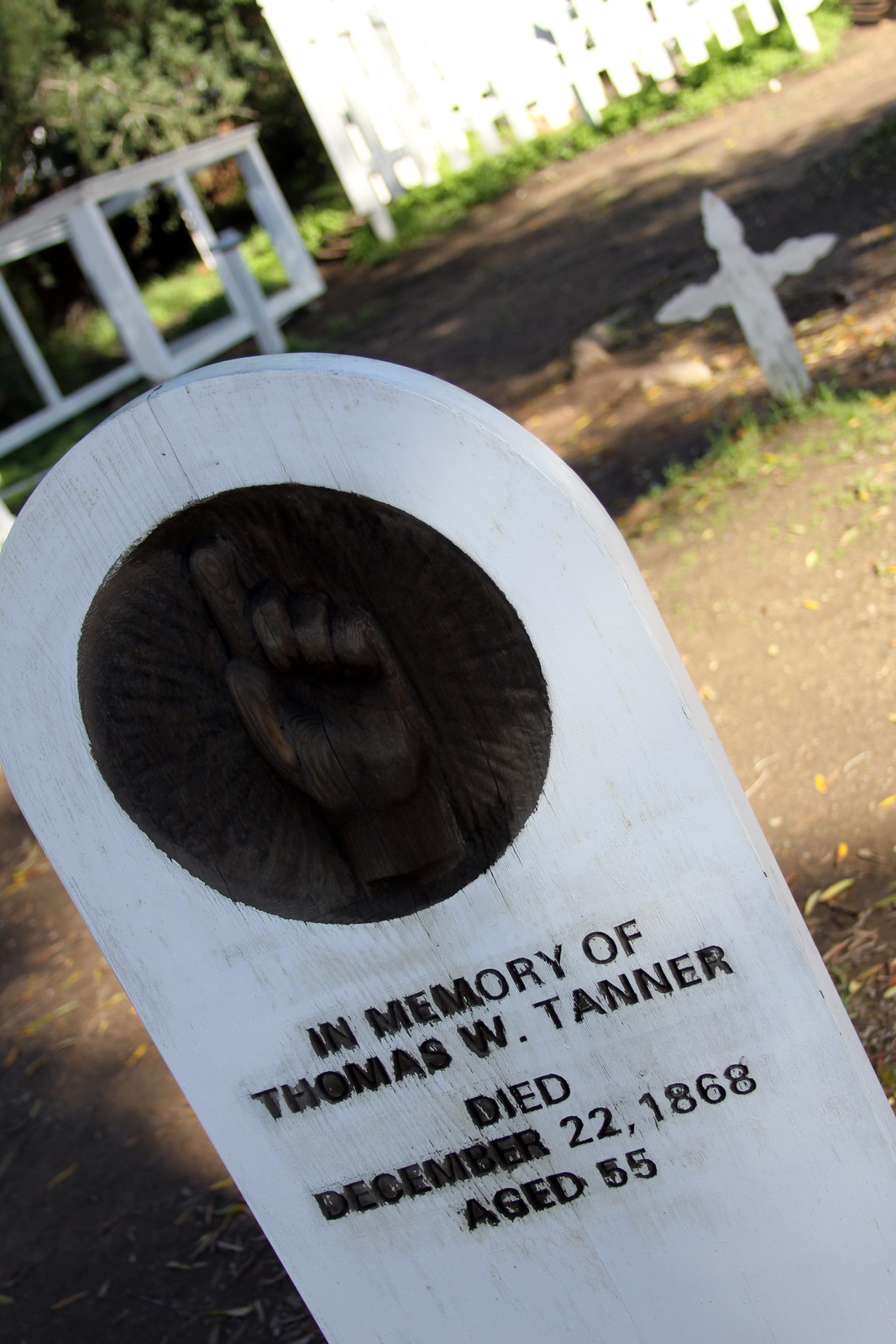The image captures a scene from a small, weather-worn cemetery, where the ground is mostly dirt with a few scattered patches of green grass. Dominating the foreground is a white tombstone, likely wooden, featuring an arched top and an inscription that reads, "In memory of Thomas W. Tanner, died December 22, 1868, aged 55," in weathered black font in all caps. Central to this tombstone is a distinct dark circle with a hand inside it, depicted with the index finger pointing upwards and the other fingers curled in, emphasizing its aged appearance. In the background, a white cross-shaped headstone stands alongside a white picket fence and a white structure. Adding to the scenery, green trees with brown stems are visible in the top left corner, providing a hint of life in the otherwise solemn setting.